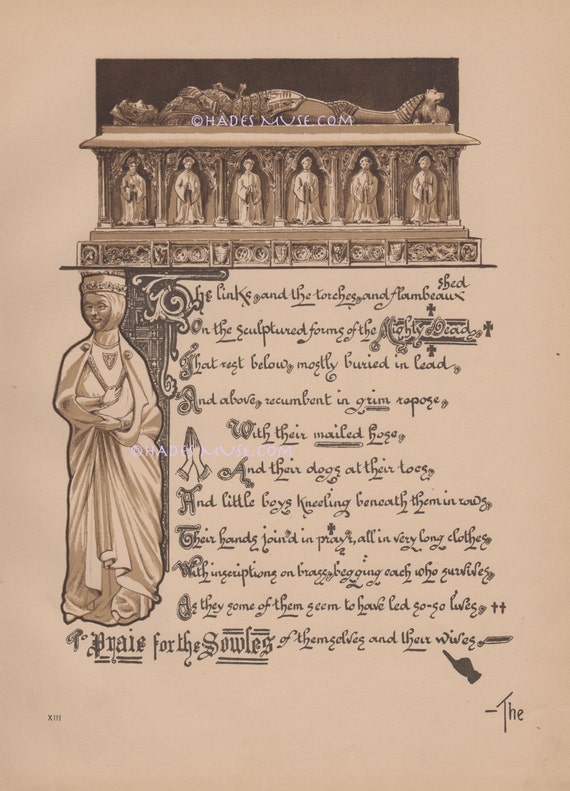This photograph captures a page from an old book, presenting a visually rich scene with a camel-brown background. Dominating the top of the page is a sarcophagus featuring a recumbent knight figure. Below this, six intricately carved statues embellish the side of the sarcophagus. On the left, an ornate statue of a figure draped in long, billowing robes is prominently displayed. The background melds lighter shades of purple and brown. The text across the page is written in an ancient and highly stylized script, with ornate and decorative letters that read, "he links and the torches and flambeau on the sculptured forms of the mighty dead." This sentence, running horizontally, is an example of the book's elaborate and historical font style, contributing to the overall antique aesthetic of the image.